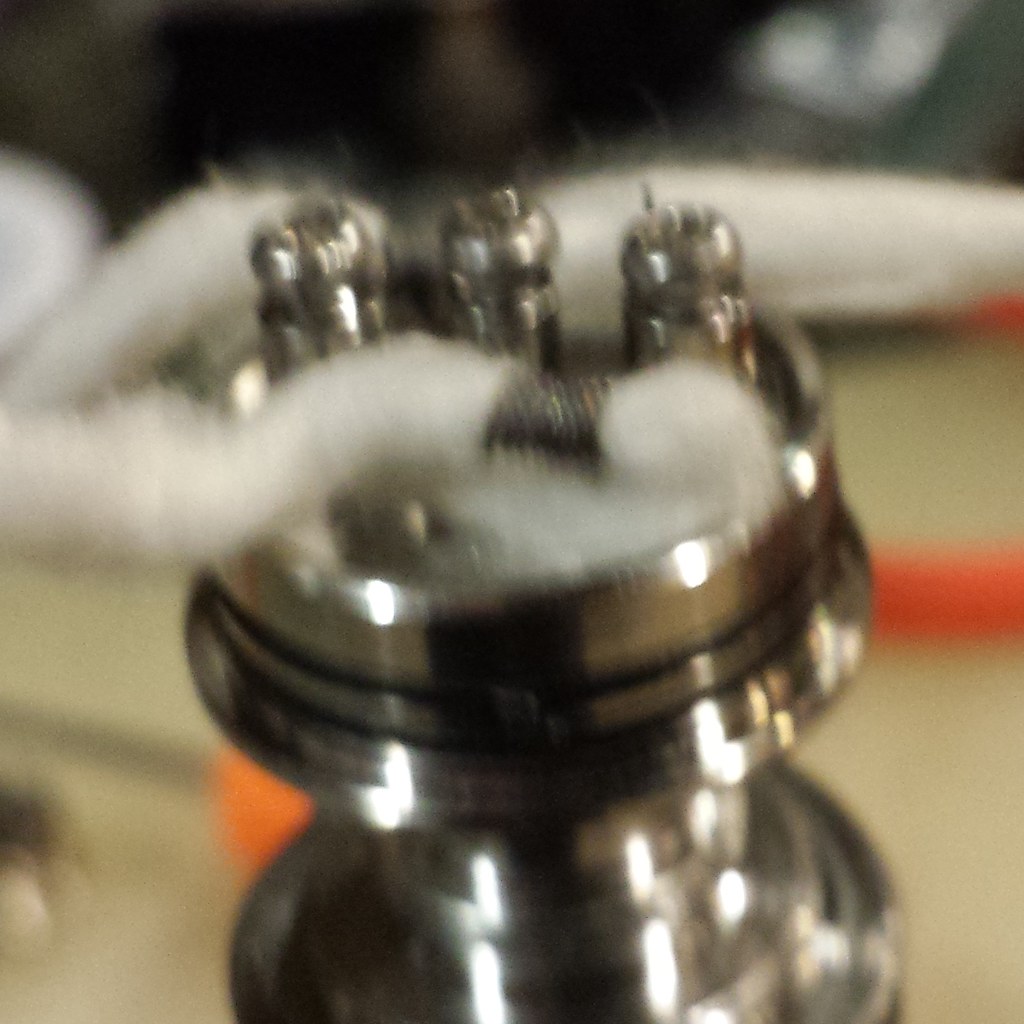This photograph depicts what appears to be a shiny, stainless steel component, blurred and difficult to identify precisely. The central object resembles a metal hub or perhaps a doorknob, possibly giving the illusion of a chess piece due to its base shape. Three shiny nozzles or prongs emerge from the top of this hub, obscured partially by what looks like white cotton batting or a piece of white yarn. This yarn-like material may be wrapped around the nozzles and extends to the back of the hub. The background remains dark and obscured, with hints of orange, adding to the overall uncertainty and mystery of the image. The scene might evoke the inner workings of a cotton candy machine, where sugar is transformed into fluffy cotton. Alternatively, it could be a part of an elaborate electrical diorama, featuring intricate metal strands and components, but the severe blurriness keeps its true nature ambiguous.